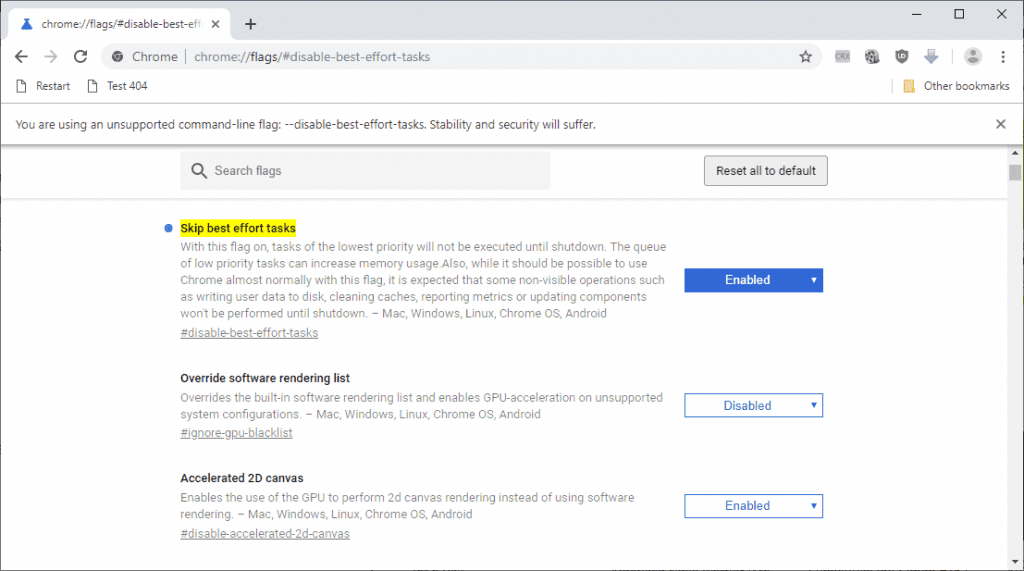Screenshot Description: 

A screenshot of the Google Chrome web browser displaying a webpage dedicated to Chrome flags. The URL in the address bar reads "chrome://flags/#disable-best-effort-tasks," indicating the user is exploring Chrome's advanced settings. The main content of the page discusses the "Disable Best Effort Tasks" flag. This flag, when enabled, prevents tasks of the lowest priority from being executed until the browser is shut down. The description highlights that while most functionalities of Chrome should operate as usual with this flag enabled, some background operations, like writing user data to disk, cleaning caches, reporting metrics, or updating components, may be delayed, potentially increasing memory usage. The compatibility of this flag across different operating systems is also noted. Below this detailed explanation, there are additional flags listed that users can enable or disable for further customization of their browsing experience.